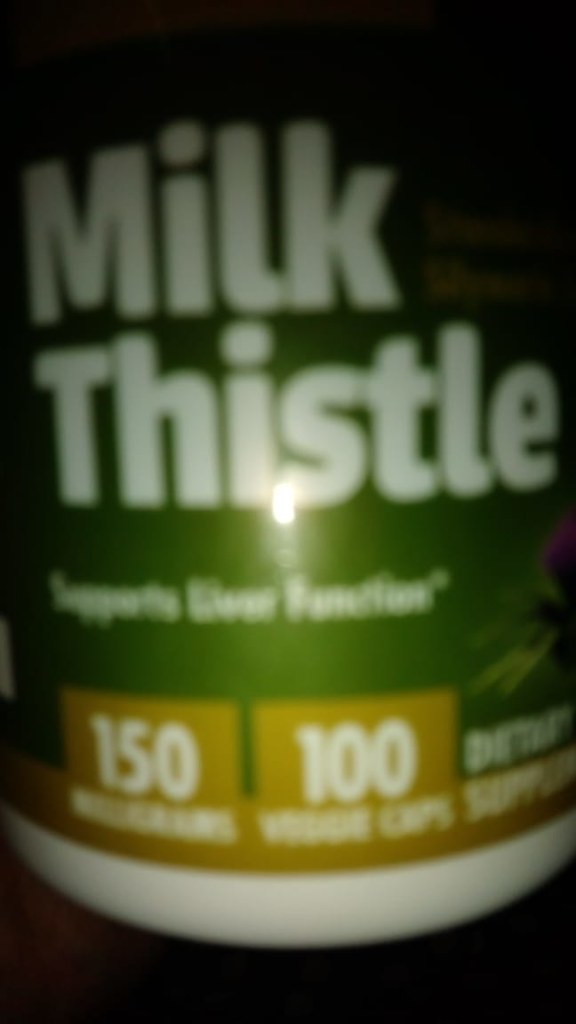The image depicts a bottle of Milk Thistle dietary supplement, designed to support liver function. The bottle features a green label with the text "Milk Thistle" prominently displayed in large, white bubble letters. Beneath it, the phrase "Supports Liver Function" is written in smaller white letters. The label also includes the number "150" at the bottom, set against a gold patch. To the side of the label, there is an illustration of a purple flower with a green stem, representing the milk thistle plant. The bottle contains 100 capsules.